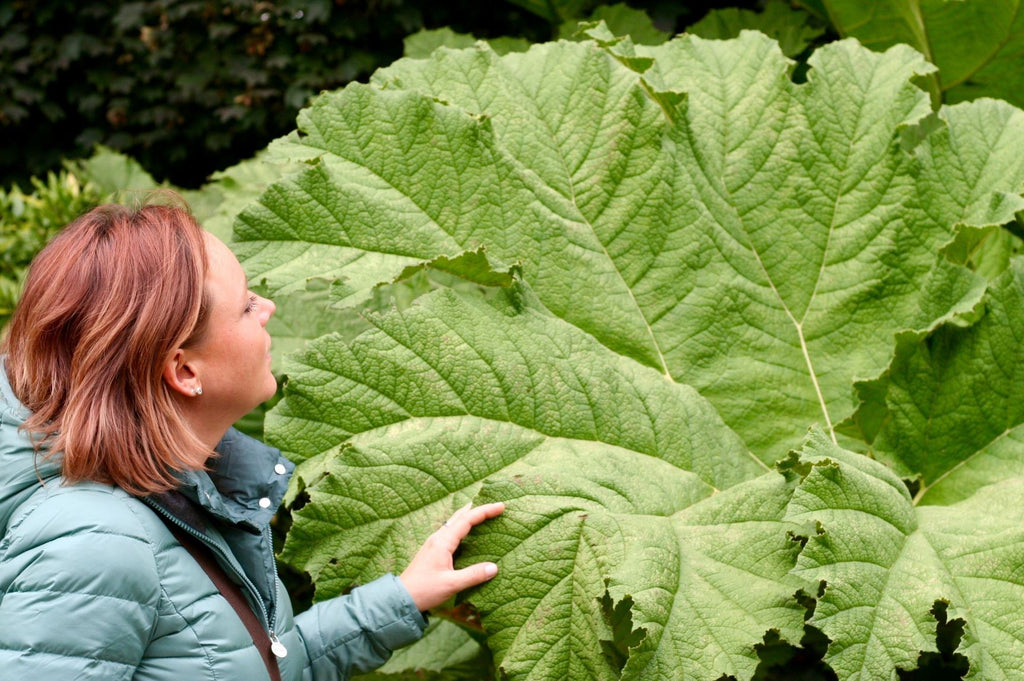In this outdoor photograph, a woman with short, slightly reddish-brown hair and a small earring is standing on the left side, facing right. She is wearing a light green, puffy jacket over a brown shirt. Her left hand is gently touching a gigantic leaf beside her. The leaf is vibrant green, almost lime in color, and has prominent veins. It is nearly as tall as the woman, with a width of around two feet. These enormous leaves dominate the right side of the image, resembling something prehistoric, perhaps like foliage ancient dinosaurs might have eaten. In the background, one can see dark green trees with normal-sized leaves, adding to the lush, natural setting. The sunlight accentuates the greenery, highlighting the impressive scale of the leaves compared to the woman.